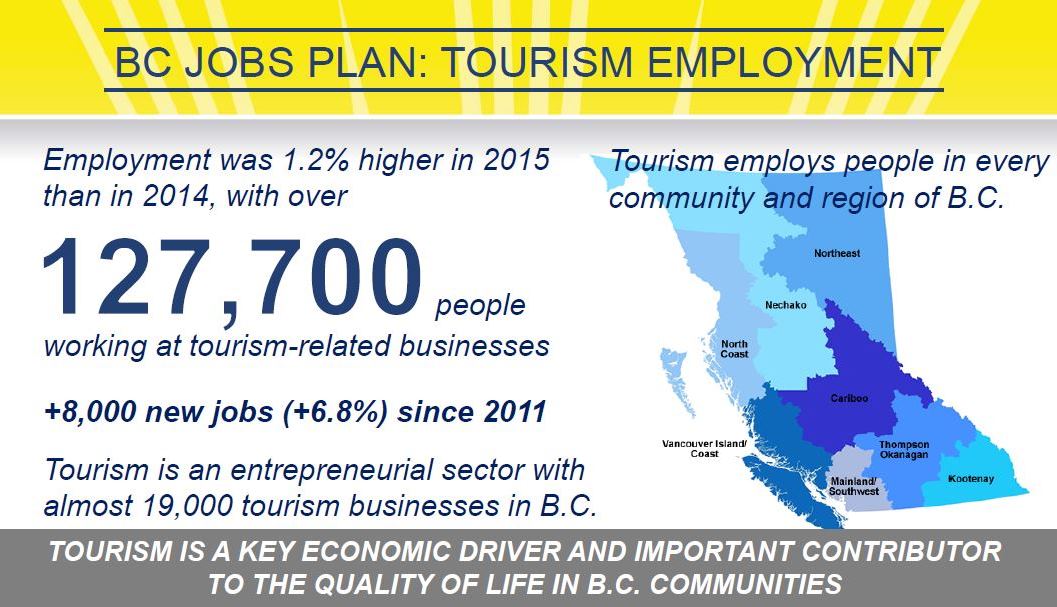The image showcases promotional material for the BC Jobs Plan focused on tourism employment. At the top, there is a cheerful yellow banner adorned with white lines resembling rays of the sun. Within this banner, dark navy blue text reads "BC JOBS PLAN: TOURISM EMPLOYMENT." Below the yellow banner, a blue line separates the header from the content below. 

The main body of the image is white, featuring a map on the right side shaded in various hues of blue. Text within this section highlights that employment in the tourism sector was 1.2% higher in 2015 compared to 2014, with over 127,700 people working in tourism-related businesses and 8,000 new jobs added since 2011, marking a growth of 6.8%. It emphasizes that tourism is an entrepreneurial sector with nearly 19,000 businesses in BC. Additionally, it states, "Tourism employs people in every community and region of BC."

At the bottom, a gray banner runs from left to right, bearing the statement in white text: "Tourism is a key economic driver and important contributor to the quality of life in BC communities."